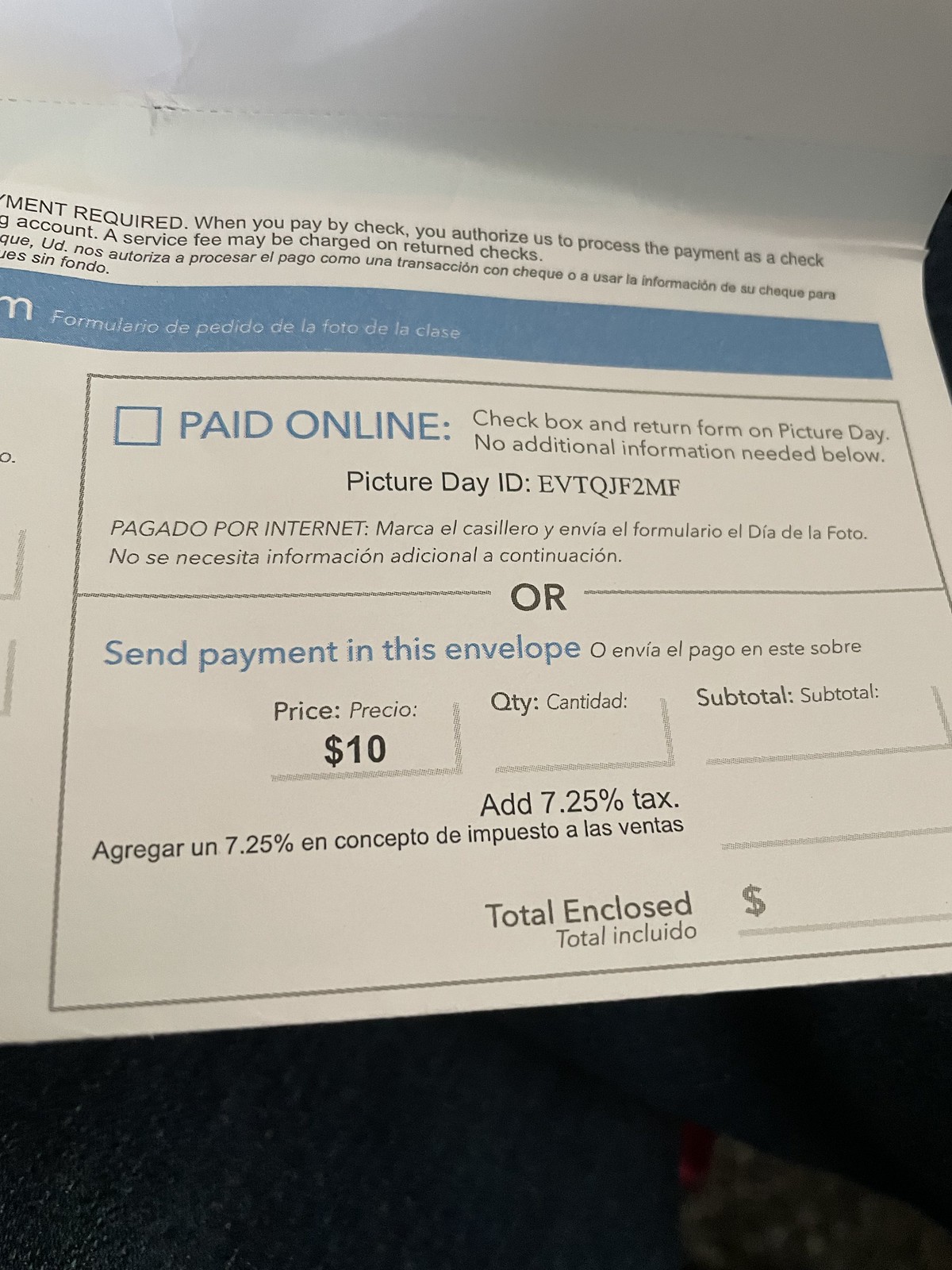This portrait-mode photograph features a white envelope designated for payment, predominantly filled with text in blue and black. The bottom 20% of the image is black, likely the surface on which the envelope rests. This envelope provides two payment options: either pay online or send payment directly in the envelope. If paying online, users must tick a checkbox and enter a picture day ID code (EVTQJF2MF), which is translated into Spanish beneath it. The other option involves sending a cash payment, specifically in denominations of $10, which happens to include an additional 7.25% tax. The envelope has fields to fill in the quantity, subtotal, tax, and total amount enclosed. The instructions likely correspond to an event known as "picture day," though the precise nature of it remains unclear. The envelope is designed to be sealed after use by folding down the top flap.